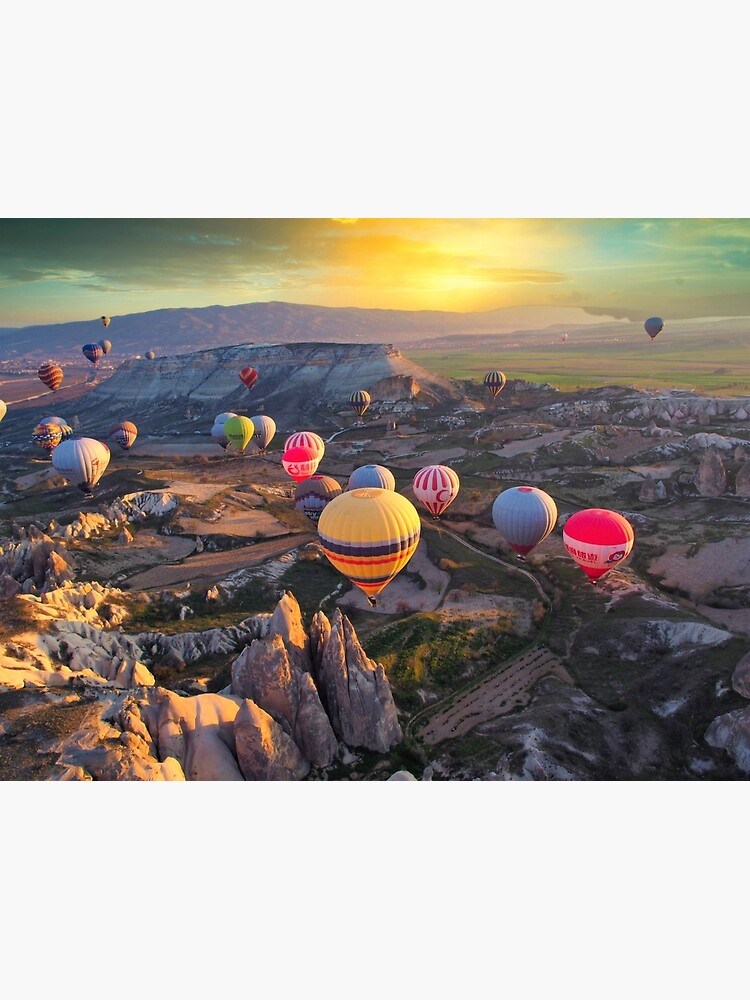This image, captured from an aerial perspective, showcases a vibrant scene of numerous hot air balloons floating gracefully over a vast, rocky landscape. The skies are adorned with a mix of bluish-gray and wispy clouds, illuminated by the setting sun. In the middle distance, an orange sun casts its warm glow over the valley, enhancing the colors of the terrain below, which features rugged rock formations interspersed with green patches of grasses and bushes.

Dominating the scene are hot air balloons of various vivid colors, including yellow, red, pink, green, blue, orange, and gray. Central to the composition is a mostly yellow balloon with distinctive blue, purple, and red markings. Nearby, a red balloon with a white stripe and a gray balloon with a red dot add to the visual diversity. These balloons appear to be more densely clustered towards the center, forming a loose line extending from right to left, with a few outliers drifting towards the horizon.

The overall impression is one of serene beauty, capturing a dynamic moment as the day transitions into evening in what is likely a renowned hot air balloon destination, possibly resembling the landscapes of Turkey. The harmonious blend of natural and man-made colors, along with the striking features of the landscape, make for an awe-inspiring aerial tableau.